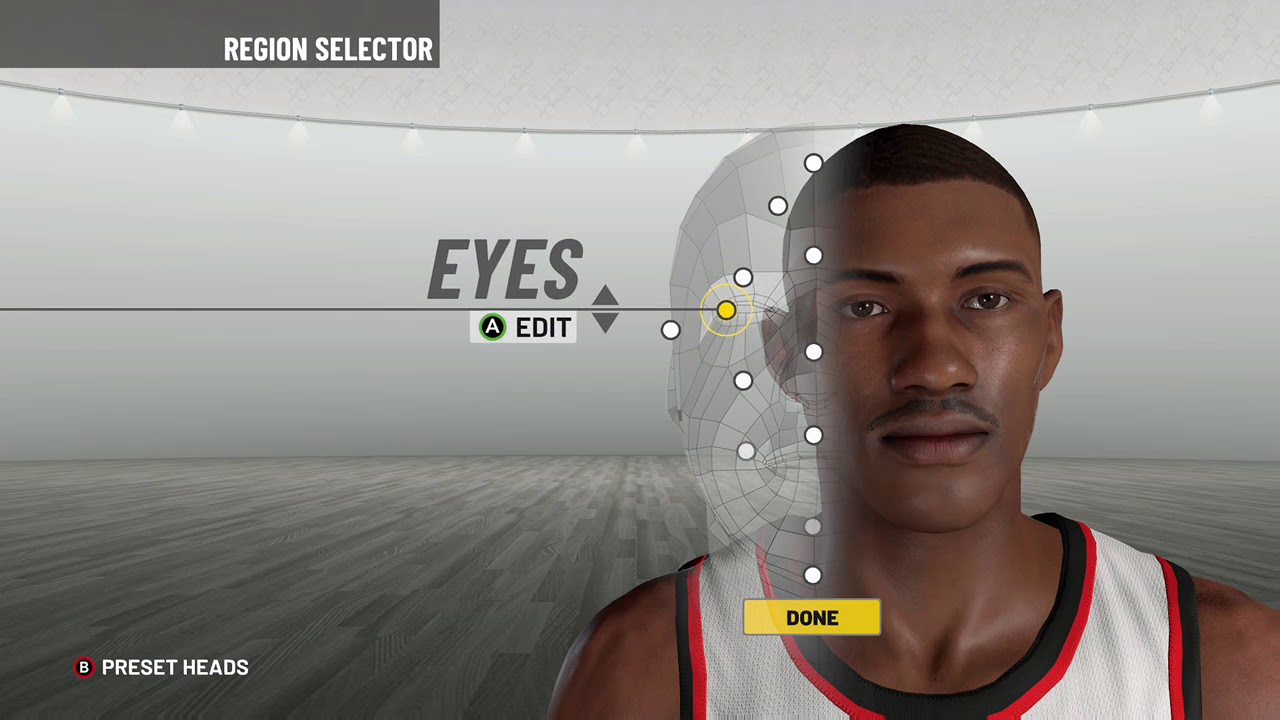**Descriptive Caption:**

A screenshot from an EA Sports NBA video game features an in-game character customization menu. The scene is dominated by a detailed 3D model of a male basketball player, an African American with short hair, a thin mustache, and brown eyes. He is wearing a basketball jersey that sports a black outline, a red middle layer, and a white core, although the specific team is not identifiable due to the lack of recognizable logos.

On the top left corner, white text against a gray background indicates "Region Selector." The ground beneath the player is covered in white tiling, adding a clean, clinical backdrop to the editing interface. The player's eye section is selected for editing, highlighted by a gray "Edit" button pointing to a yellow circle on the 3D model, suggesting active editing parameters. At the bottom of the screen, there is a "Done" menu option for finalizing changes.

This interface seems typical of EA Sports' NBA video games from the past few years, showcasing their robust character creation tools. The bottom left corner features a prompt for the "B" button, indicating a potential exit or back function, common in console gaming interfaces.